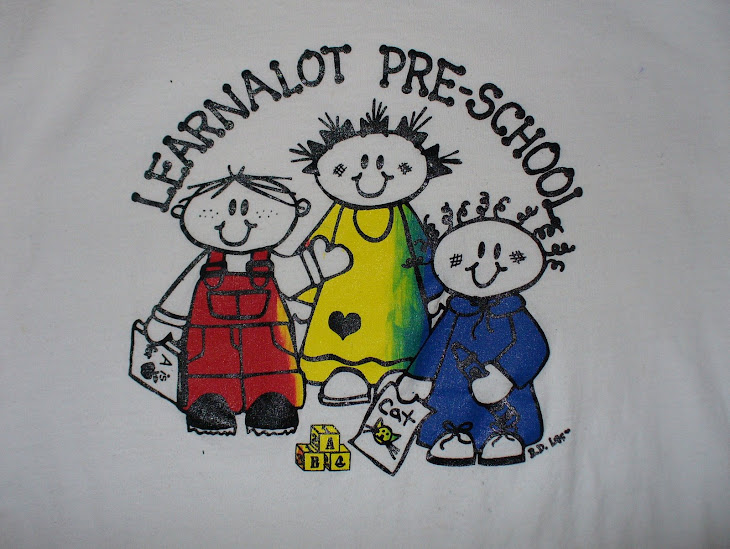The image is an advertisement for Learn A Lot Preschool with a white background. At the center is a light gray rectangle with black text that reads "Learn A Lot Preschool" in an arched rainbow shape. Below the text are black line drawings of three children. The first child on the left is wearing red overalls and black shoes, smiling while holding a book with an A and an apple in one hand and waving with the other. The middle child, a girl, is smiling and dressed in a yellow and blue dress with a heart on the lower left corner. She has black hair styled in bows. The third child, with black curly hair, is wearing a blue hoodie and white sneakers; this child is holding a piece of paper with a drawing of a cat and the word "cat" on it. In front of the children are three building blocks with the letters A, B, and a sailboat. In the bottom right corner of the image, there is additional text that reads "RD Loss."